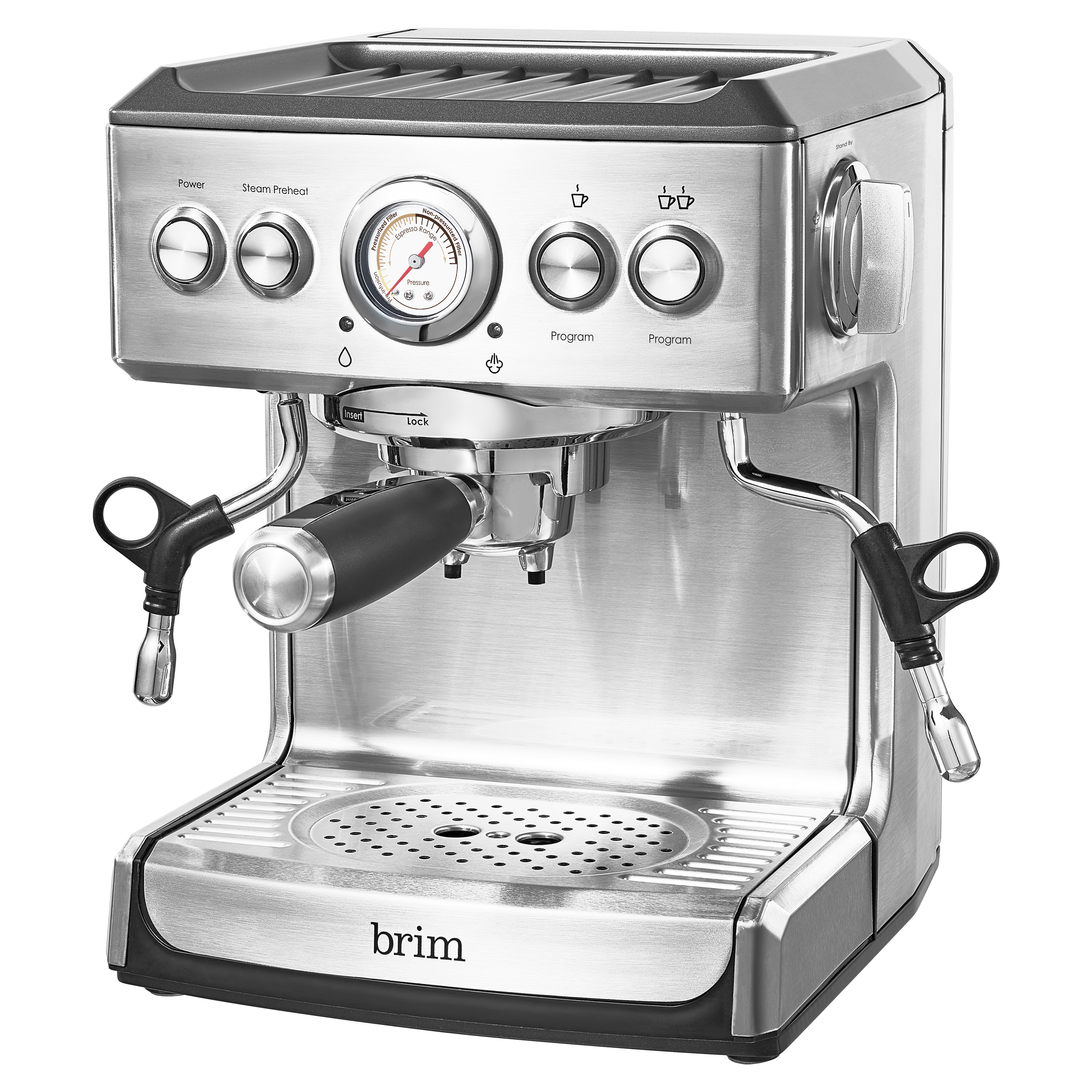This detailed product image prominently features a high-end espresso machine, specifically a Brim brand model. The device is crafted from stainless steel, giving it a sleek and shiny appearance, indicative of a new and clean condition. Positioned at a diagonal angle, the photo showcases the front, side, and top of the machine, which occupies almost the entire frame, emphasizing its significant presence. 

The espresso machine's main body is a lustrous silver metallic with various accents in black, white, red, and clear. The top surface is black, complemented by a black base made of plastic. Notable details include a central black handle used for inserting the coffee grounds, and milk frothing nozzles extending from either side, each adorned with black handles.

The front panel is adorned with multiple buttons and dials, including a power button, a steam preheat button, and two programmable buttons labeled with single and double coffee cup icons. Additional indicators feature symbols like a water droplet and a cloud, likely representing steam and water functions. At the bottom of the front panel, the brand name "Brim" is displayed in lowercase black text against the stainless steel background.

This meticulously photographed image, set against a plain white backdrop, highlights the machine's sophisticated design and functional elements, making it suitable for a retail setting like a kitchen appliance sales site.